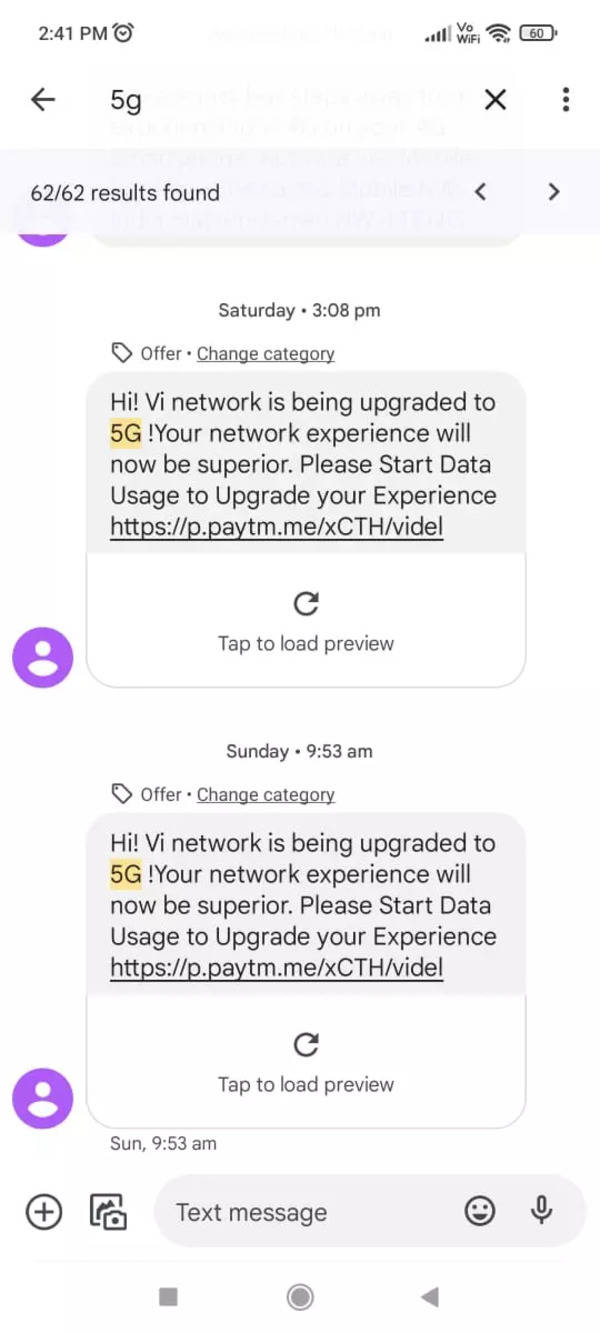This is a detailed screenshot captured from a smartphone at 2:41 p.m., visible in the upper left-hand corner. The battery icon in the upper right-hand corner indicates a 60% charge. At the top of the screen, a left-facing arrow and the text "5G" are displayed. Just below, a light gray bar shows "62 of 62 results found."

The screenshot contains two messages. The first message, timestamped Saturday at 3:08 p.m., reads: "Offer, Change Category, Hi, VI Network is being upgraded to 5G." The phrase "5G" is highlighted in yellow. The message continues, "Your network experience will now be superior, please start data usage to upgrade your experience." A URL address follows this text, accompanied by a small white box that says, "Tap to Load Preview."

The second message, similar to the first, is timestamped Sunday at 9:53 a.m. At the bottom of the screen, there's a text entry box labeled "Text Message."